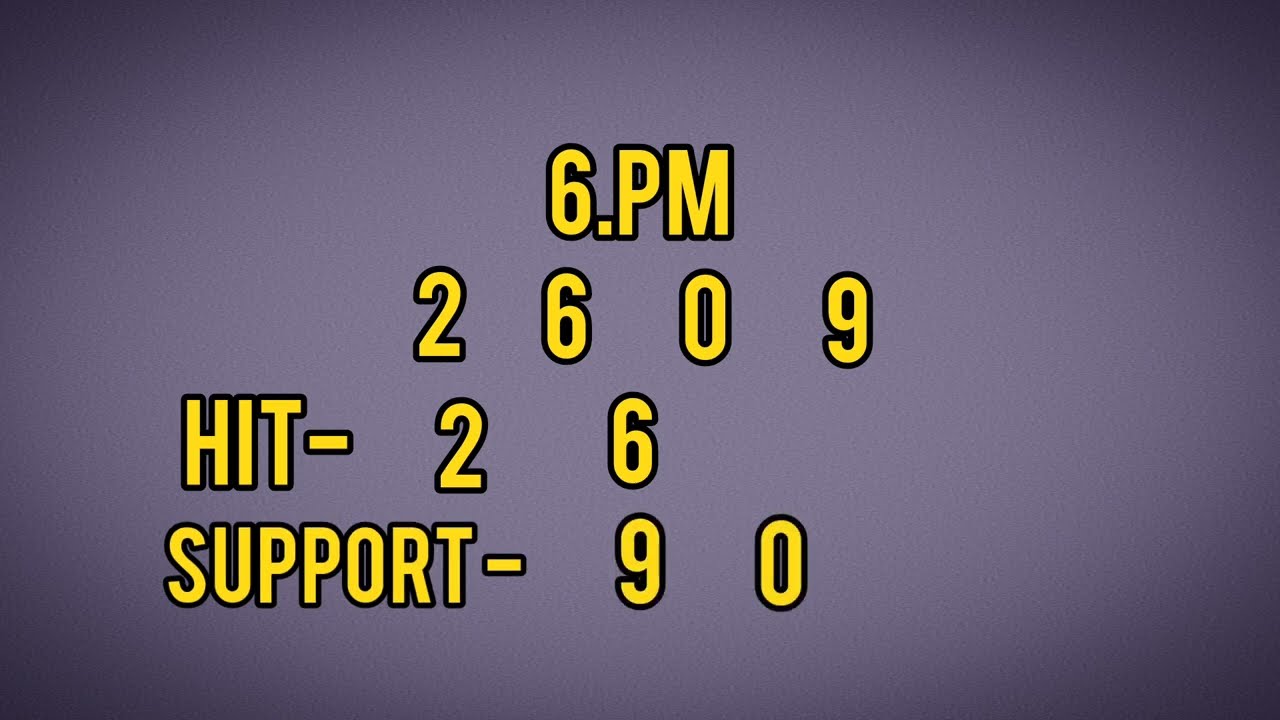The image features a text-based layout reminiscent of a scoreboard, centrally aligned on a gray background that transitions from dark at the edges to a lighter shade in the middle. Dominating the visual are large yellow numbers and letters outlined in black. At the top center, "6.PM" is prominently displayed. Directly beneath that, in the same bold font, the sequence of numbers "2 6 0 9" is spaced widely apart. Below this sequence, slightly to the left, reads "HIT-2 6," with generous spacing between the characters. At the bottom center, the word "SUPPORT-9 0" is similarly formatted. The overall composition is simple yet striking, with the interplay of yellow, black, and varying shades of gray.